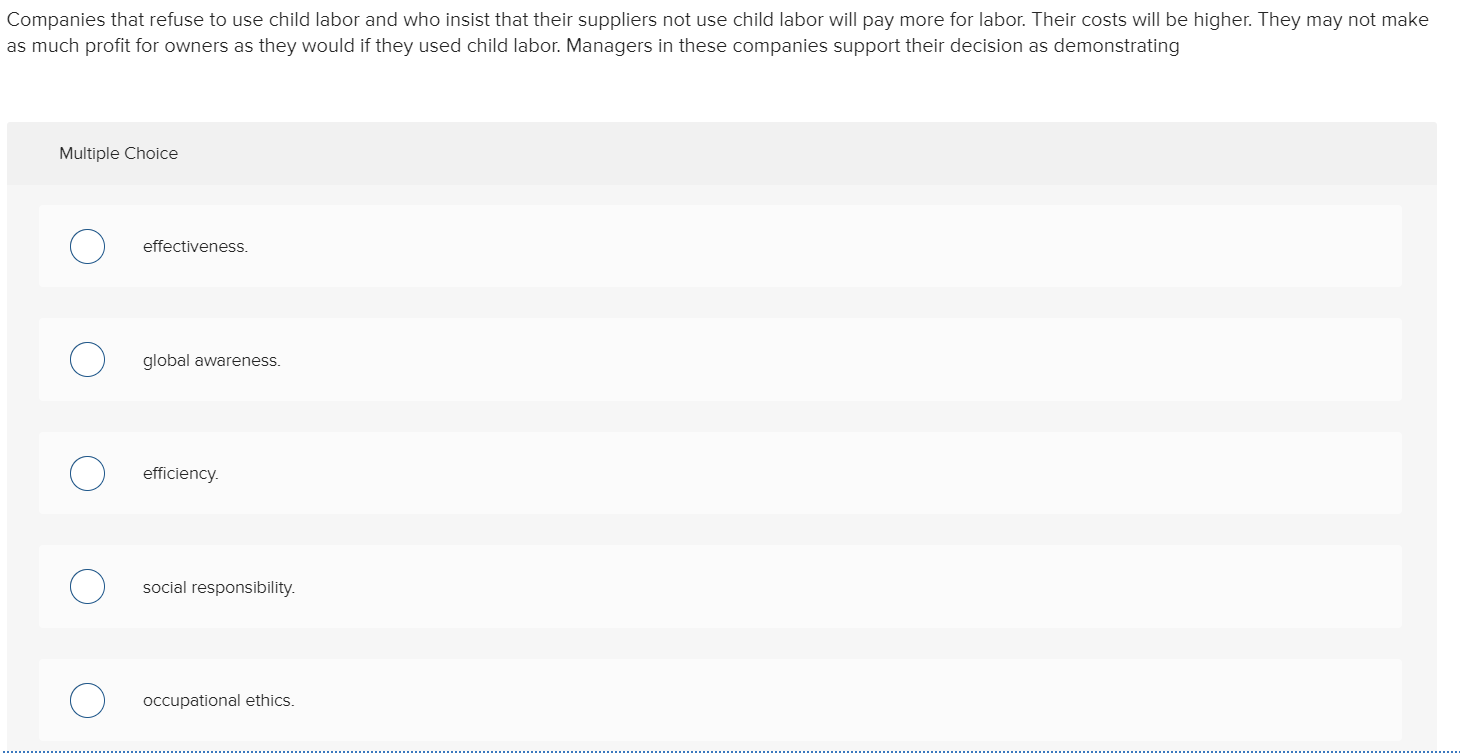This image features a screenshot of a test question centered on business ethics. At the top, the question discusses companies that refuse to use child labor and insist their suppliers do the same. These companies recognize that such ethical practices will increase labor costs and potentially reduce profits compared to those who exploit child labor. However, managers in these companies support their decision, believing it demonstrates a significant corporate value.

Beneath the question, a gray box containing multiple choice options is displayed. The box is labeled "multiple choice" at the top. Below this label, there are circular radio buttons next to each option, allowing selection. The listed options are: "effectiveness," "global awareness," "efficiency," "social responsibility," and "occupational ethics." The overall scene emphasizes a consideration of ethical practices within business operations and the values upheld by companies committed to social responsibility.